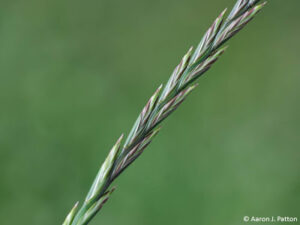This high-definition, detailed, landscape-oriented photograph by Aaron I. Patton captures the essence of nature's simplicity and intricacy. The central focus is a light green plant, potentially a special type of grass or plant stalk, that diagonally arcs from the bottom left toward the top right of the image. Its delicate blades wrap around the stem, some displaying budding flowers with a hint of purple. The background, a deep green blur, suggests a lush surrounding that remains indistinct, emphasizing the plant's vivid clarity. The lower right corner bears a white watermark crediting the copyright to Aaron I. Patton. The photograph, rendered in photographic representational realism, draws viewers into the natural serenity it depicts.